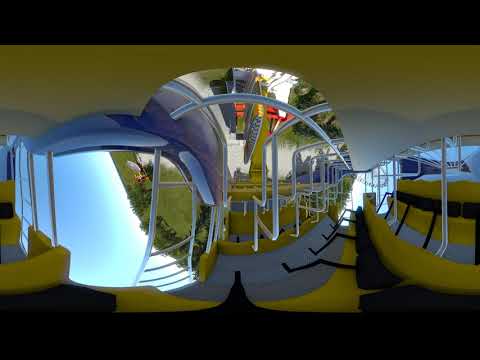This color photograph in landscape orientation uses a fisheye lens and a distorted barrel filter effect to create a unique visual. The center of the image features a structure with bluish-purple elements supported by cylindrical poles. The top and bottom 5-10% of the image are occupied by horizontal black bars. Around the central structure, areas of green grass, resembling putting greens, appear on the left and right. The background displays a white wall, possibly from a building, and an orange, arched roof. Sunlight creates black shadows from some of the white, cylindrical poles, which also feature light turquoise areas underneath the overhangs. The image is divided into three segments: the left side shows white ladder bars tilted sideways against a blue sky; the middle segment focuses on the main structure with overhead bars and green grass; and the right side presents a portion of the structure with visible white bars and landscape elements. Despite the complexity and lack of identifying text, the photograph’s distinctive elements and colorful distortions suggest a theme of photographic representationalism.